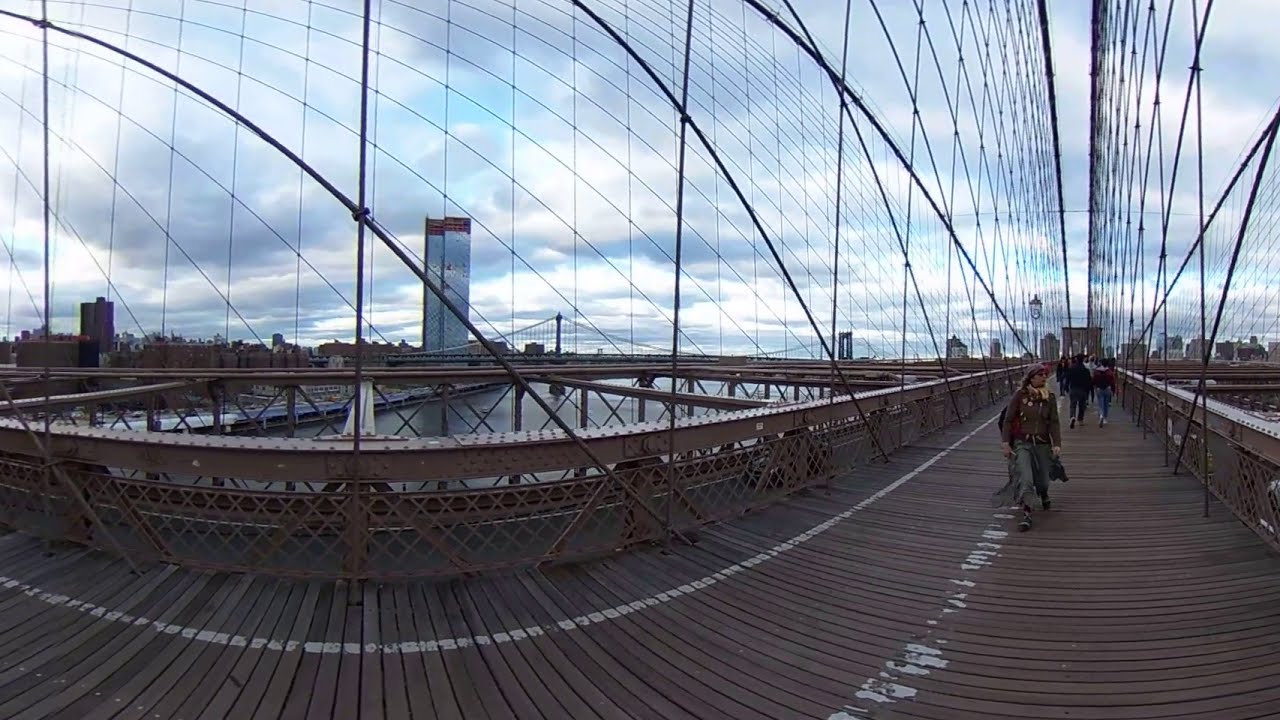This photograph, likely taken with an ultra-wide-angle or fisheye lens, captures a dynamic urban scene of a pedestrian suspension bridge on a partly cloudy day, possibly in Vancouver, Washington. The bridge, built from horizontal wooden slats and divided by white lines for both foot traffic and bicycles, spans over a shimmering waterway. The image features several pedestrians, with the most prominent figure wearing pants, a scarf, glasses, a hat, and carrying a backpack. The ultra-wide lens causes a dramatic curvature of the bridge, especially noticeable on the left side, enhancing the sense of depth and distortion. This curved structure is lined with steel girders and cables that stretch up to the suspension lines overhead. On the far left of the image, reflecting the partly cloudy sky, stands a mirrored skyscraper, while other buildings and additional bridges can be seen in the distance, contributing to the urban backdrop. The scene is bustling with movement and captures a vibrant slice of city life.